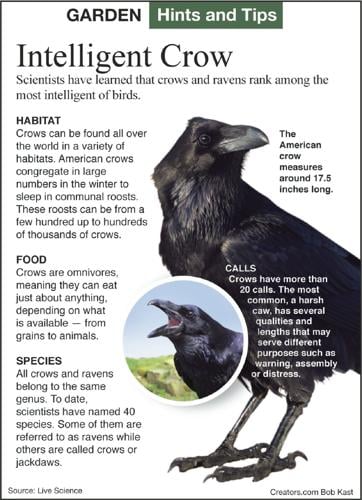The page, likely from a magazine or a book, is titled "Garden Hints and Tips" with "Hints and Tips" in white letters on a green background and "Garden" in black. The layout features a main headline “Intelligent Crow” in large letters, with the text explaining that crows and ravens are among the most intelligent birds. The focal point is a prominent black crow image on the right side. Below the headline, detailed sections provide insights into the crow's habitat, food, and different species. In the center, there's a circular insert with a blue background and green grass, depicting another crow with its beak open, facing left, emphasizing the crow's communicative abilities. The insert highlights that crows have over 20 distinctive caws used for communication like warnings, assembly, and distress signals. The entire page is primarily in black and white except for the crow images and the 'Hints and Tips' header, which are in color. The bottom corners feature credits: “Creators.com, Bobcats” on the right and “Source Life Science” on the left.